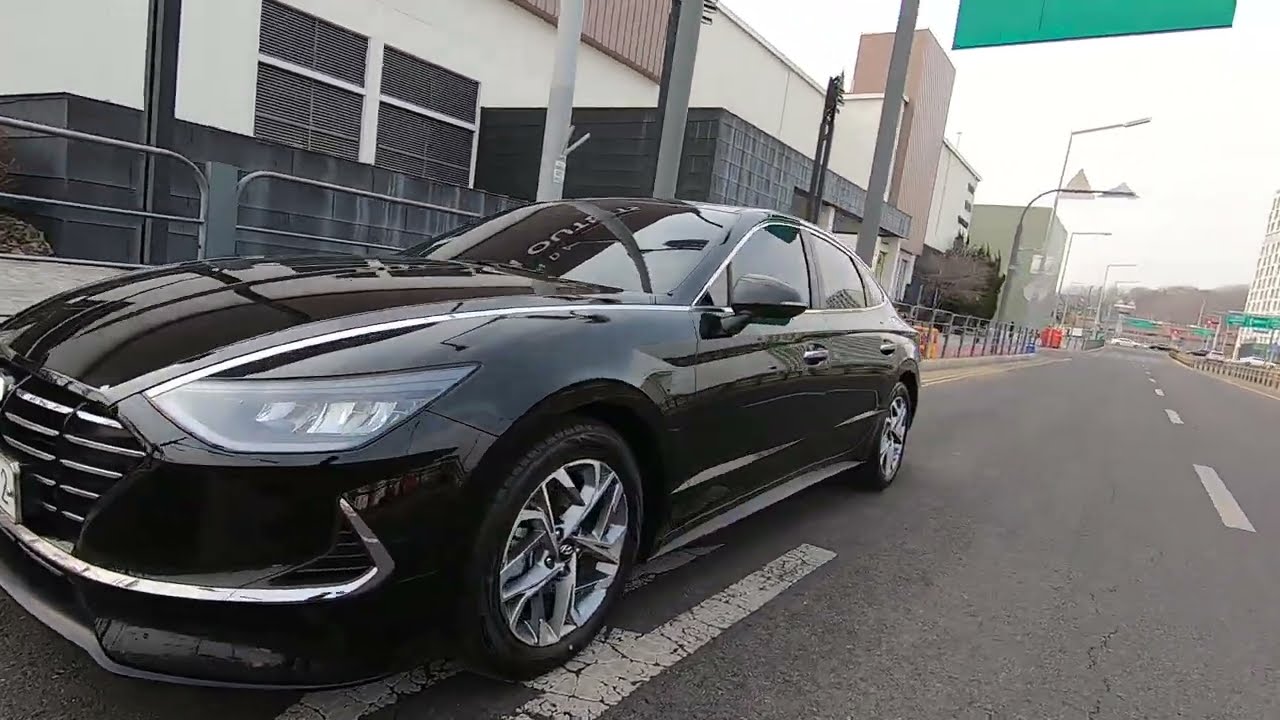The image is a horizontally aligned rectangular close-up of a shiny black sedan with sporty silver rims, parked on the left side of a two-lane street. The street, which features an older gray surface with a white dashed center line, extends across the lower right side and left side of the photo. Surrounding the car, the scene showcases urban elements: on the left, there is a prominent two-story building with a bottom section featuring black details and a mostly white stone upper part, accented with brown trim near the roof. Partially visible in the background on the left are more office buildings that have modern white, brown, and black facades. 

To the right, barely in the frame, stands another tall white building, implying a bustling cityscape. In the upper right-hand corner, a green street sign's backside is visible, with additional green directional highway signs fading into the background further along the street. The scene also includes street lights lined up behind the car along the curb and some orange construction cones in the foreground. The sky overhead is overcast, casting a diffuse white light over the entire scene, emphasizing the car's sleek and reflective surface.